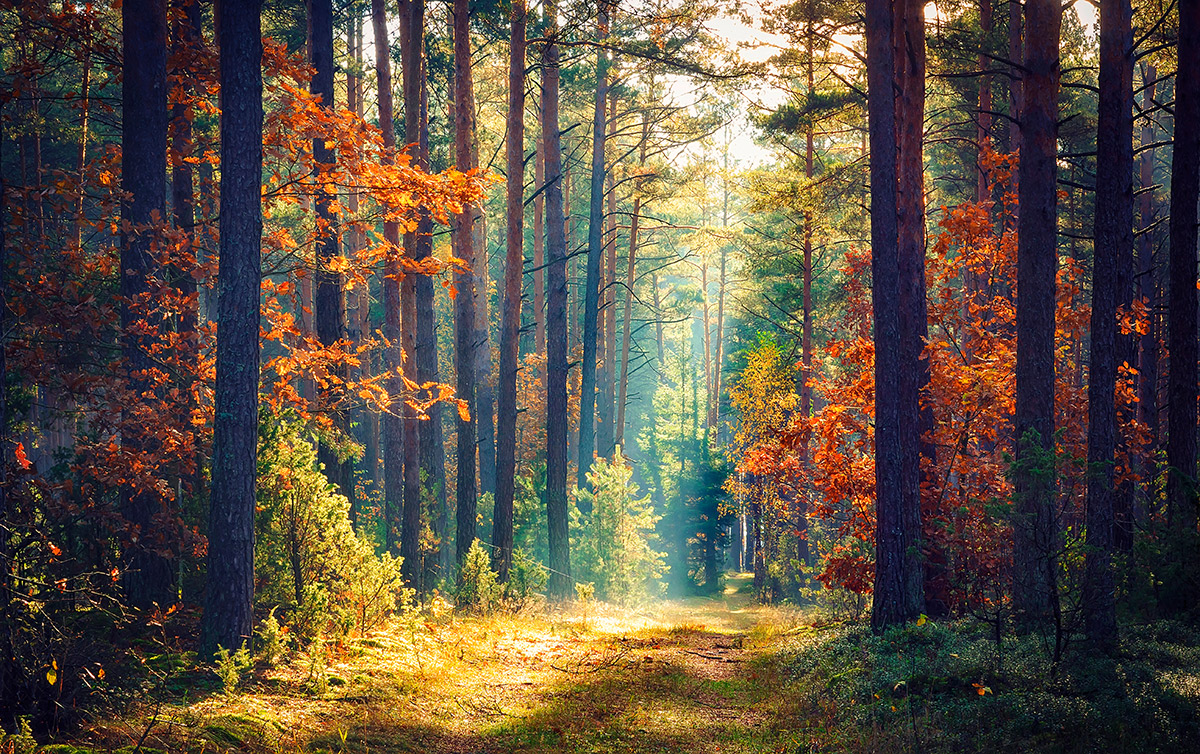The image depicts a serene forest scene, possibly a painting or a digitally rendered artwork, with an inviting, grassy path meandering through lines of tall, mature trees intermixed with younger, smaller ones. The towering trees form a canopy, some reaching heights where their tops extend beyond the frame. Along the trail, which appears intentionally maintained with evenly cut grass, sunlight streams through the gaps in the foliage, casting dappled shadows and illuminating patches on the forest floor.

The forest is predominantly green, but a seasonal transformation is evident as several trees near the ground sport vibrant orange, yellow, and red leaves. This seasonal shift contrasts beautifully with the pervasive greenery, hinting at autumn's onset. The scene is bathed in a golden hue where the sunlight meets the ground, enhancing the tranquil and inviting atmosphere. The fringes of the path are marked by darker shades, where the dense clusters of leaves prevent sunlight from penetrating, maintaining a rich, dark green tone. A sliver of blue sky is visible in the upper center, confirming the scene is set in daylight. This picturesque forest path, embedded in a mix of towering pines and deciduous trees, evokes a sense of peace and natural beauty.